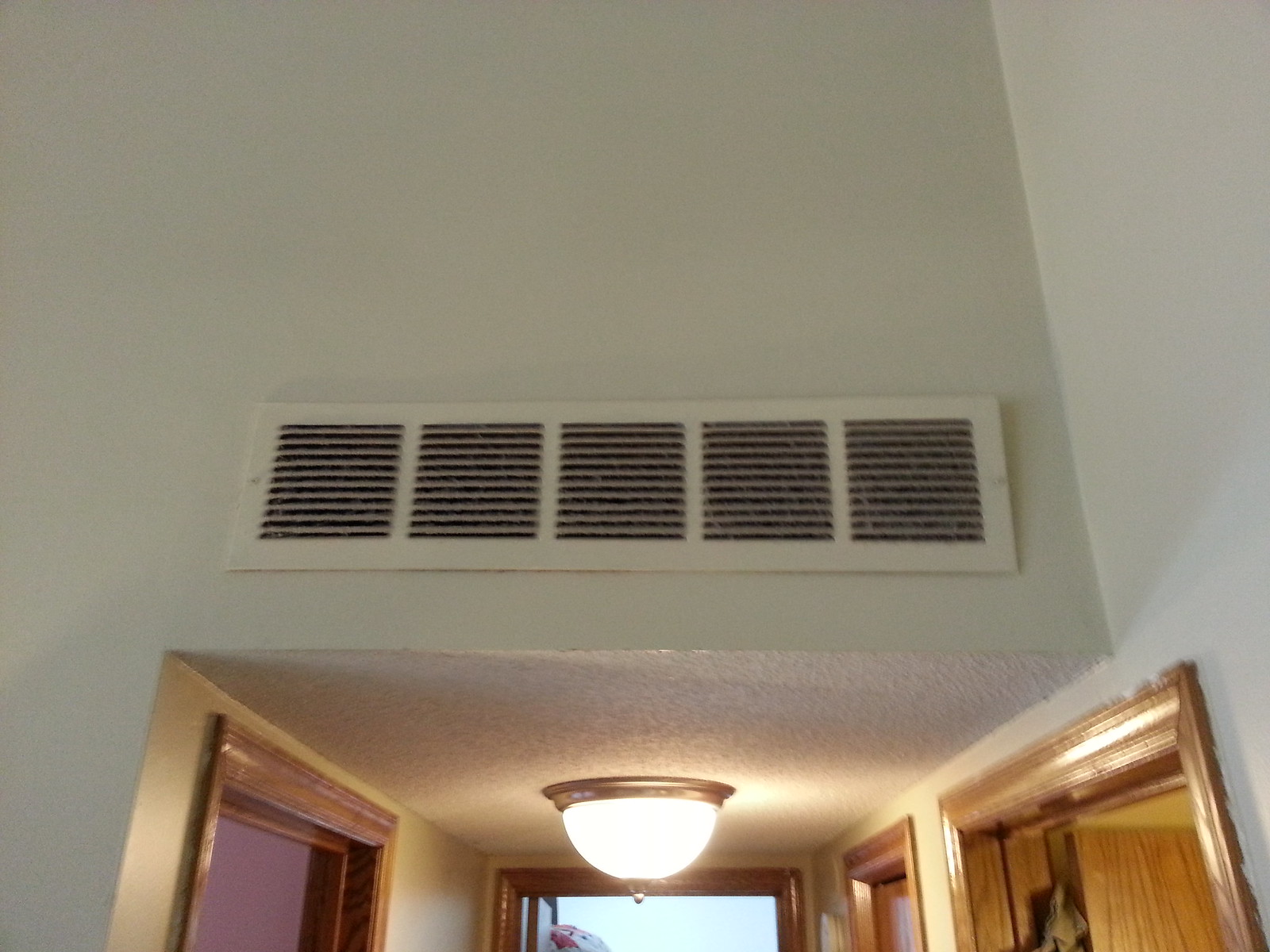This image depicts the interior of a hallway with a medium gray wall at the top of the frame. Centered on this wall is a horizontal vent featuring five square registers, each with intricate line patterns, spanning approximately six to eight inches in length. Below the vent on the ceiling hangs a bright, white pendant light, shaped like a semi-sphere with a central button. This light illuminates the hallway, which contains four doorways with natural, brown wooden frames. One doorway, located in the back right corner, is closed, while another adjacent to it is halfway open, revealing a brown door. The remaining doorways on the left and right are open; the former appears to lead into a room with a pink wall, and the latter shows a hint of blue light within. The vent itself looks a bit dusty, suggesting it might need some cleaning. The overall composition indicates a well-used, possibly multi-level home space.